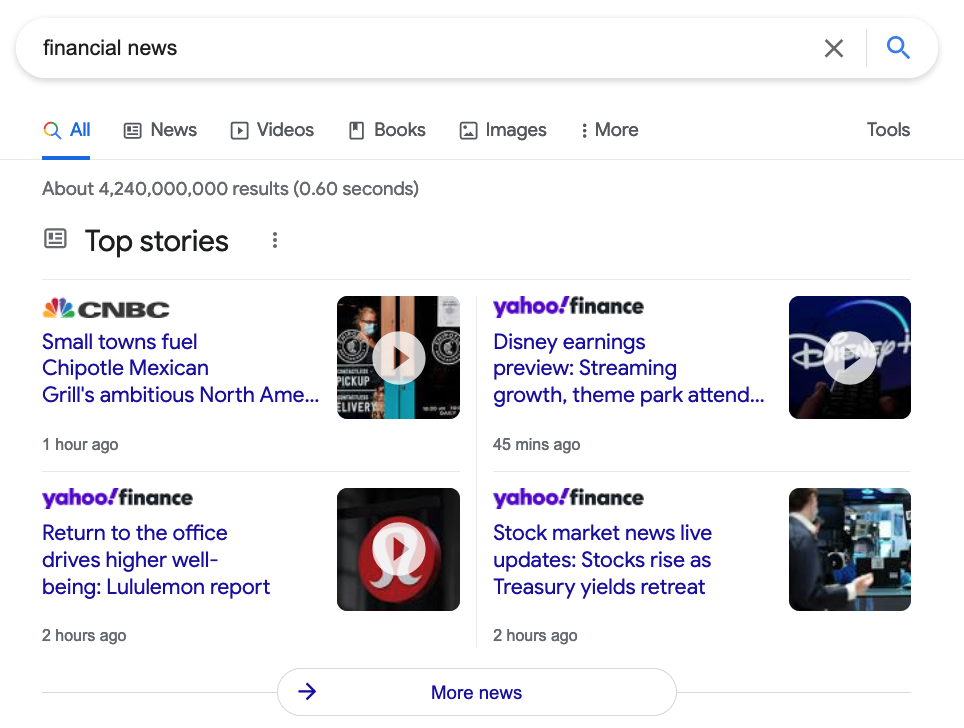Displayed on a typical Google search page, characterized by its plain white background and blue hyperlinks, the screen shows Google Financial News with approximately 4.2 billion results. At the top, prominent headlines from various reputable financial sources are featured. CNBC's headline discusses how small towns are fueling Chipotle Mexican Grill's ambitious growth. Yahoo Finance presents multiple stories, including a Disney earnings preview and an article on the return to office trends driving higher well-being. Another exclusive Yahoo Finance report covers Lululemon's performance, accompanied by the company's logo, while their stock market news update includes a photo of a man at the New York Stock Exchange. Additionally, a 'More news' button at the bottom signals the availability of further updates. The page also permits the user to search by categories such as news, videos, books, and images, with a tools button in the top right corner for modifying search settings. Three of the headlines include video content, enhancing the multimedia news presentation.